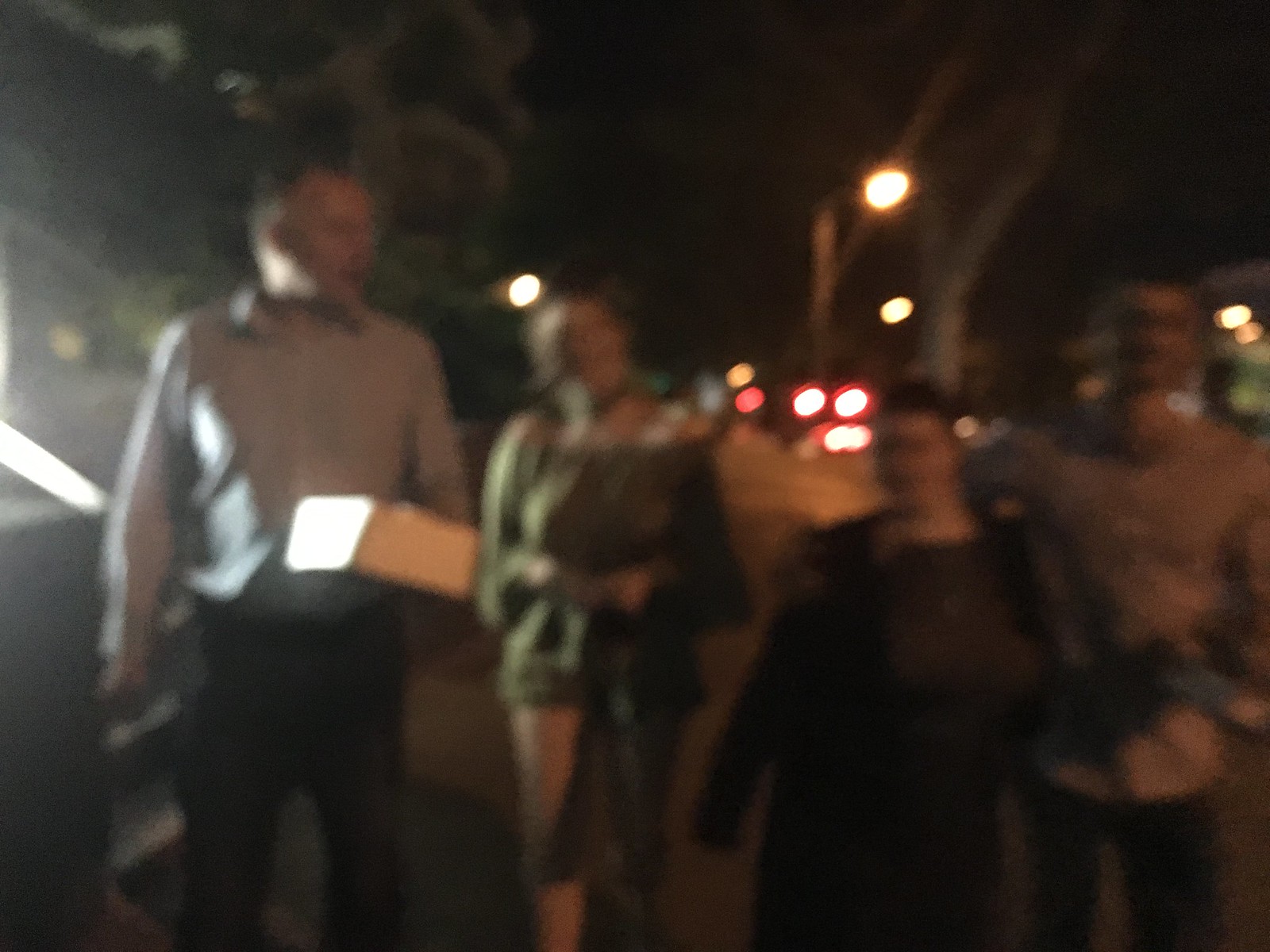This is a blurred, nighttime color photograph taken outdoors, depicting four people walking down a sidewalk towards the camera. The tallest man on the left is holding a white box, possibly containing a cake or leftovers from dinner. He wears a blue, long-sleeved dress shirt, black pants, and might have glasses, although it's difficult to see due to the blurriness and dim lighting. He appears to be middle-aged, with short hair, possibly a buzz cut, and he's looking left as his right hand dangles by his side.

Next to him is a woman wearing an off-the-shoulder, long-sleeved green blouse with shorts. She has blonde hair and may be wearing a scarf. To her right is another woman who is shorter and wearing a purple or brown dress with a black overcoat or jacket. Her hair seems to be pulled back, and she's slightly heavier set.

Beside her, on the far right, stands a man with his arm around her shoulder. He is dressed in black pants and an untucked white or blue and white button-up shirt. He might be wearing glasses and has a mustache.

They are walking on a dimly lit sidewalk, with street lamps, electrical lines, and trees visible in the background. A staircase to the left is illuminated, creating a soft glow that contrasts with the overall grainy and out-of-focus nature of the photograph.